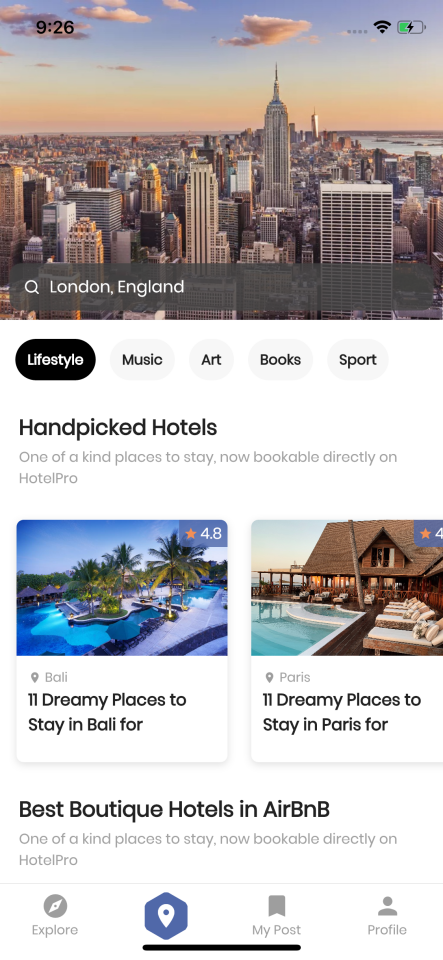Screenshot of a mobile phone displaying a cityscape background at sunset, potentially showcasing London's skyline. In the top left corner, the time "9:26" is indicated in black text. On the top right, icons show a connected Wi-Fi symbol and a battery indicator with about half charge, featuring a lightning bolt and a green bar.

Below the city image, a gray rectangular search bar with rounded corners reads "London, England" in white text, accompanied by a white magnifying glass icon on the left. Directly beneath the search bar, five navigation buttons are aligned horizontally: Lifestyle (highlighted in black), Music, Art, Books, and Sports (all in gray).

Further down, a headline in black text reads "Hand-picked hotels," followed by a subtitle in gray text stating "One of a kind places to stay, now bookable directly on Hotel Pro." Displayed below are two hotel options with images: one for Bali and one for Paris. The text under the image for Bali reads "11 dreamy places to stay in Bali," and for Paris, it reads "11 dreamy places to stay in Paris." Additional informative text in black states "Best boutique hotels in Airbnb," and in gray, it reiterates "One of a kind places to stay, now bookable directly on Hotel Pro."

At the very bottom, four navigation icons are evenly spaced: Explore, a map icon, My Post, and Profile.